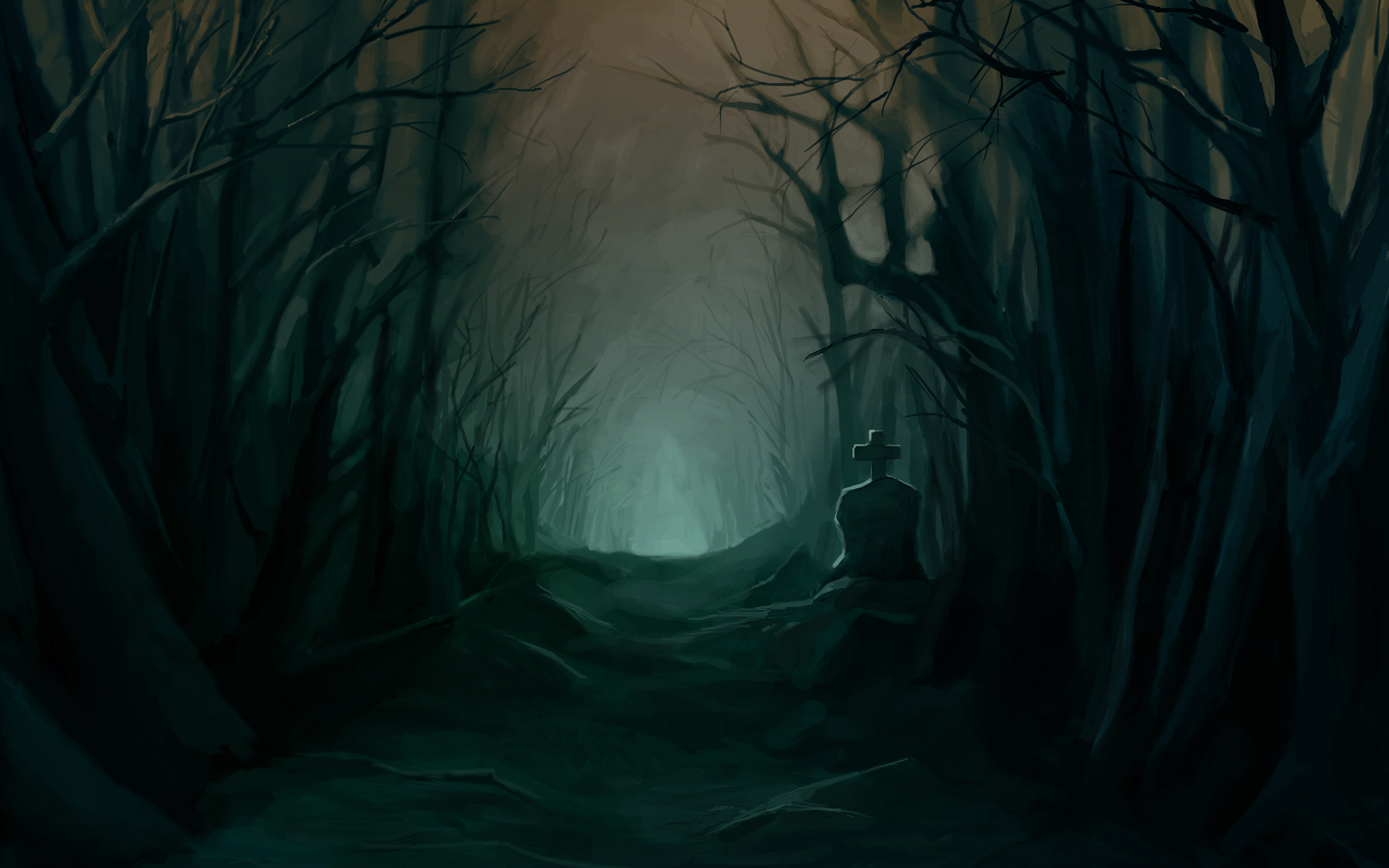This painting, evocative of a dark and haunting scene, is set outdoors at night, capturing the viewer from the vantage point of someone standing at the edge of a dense forest. The foreground is shrouded in darkness, highlighting the eerie atmosphere of the setting. To the right, silhouetted trees devoid of leaves stand ominously, while to the left, smaller, similarly dark tree silhouettes create a sense of depth and foreboding. Between these rows of trees, a distinct headstone with a cross stands solemnly, adding to the spooky ambiance.

Central to the composition is a mysterious light blue triangle that illuminates the middle of the painting, drawing the eye towards its ethereal glow. Slightly to the right of this central light, a figure can be seen in silhouette, possibly seated and wearing a hat, adding an element of intrigue and human presence amidst the spectral light. The branches and trunks of the trees, all in silhouette, weave a dark tapestry that seems to hide the secrets of the night, further enhancing the painting's haunting and enigmatic mood.